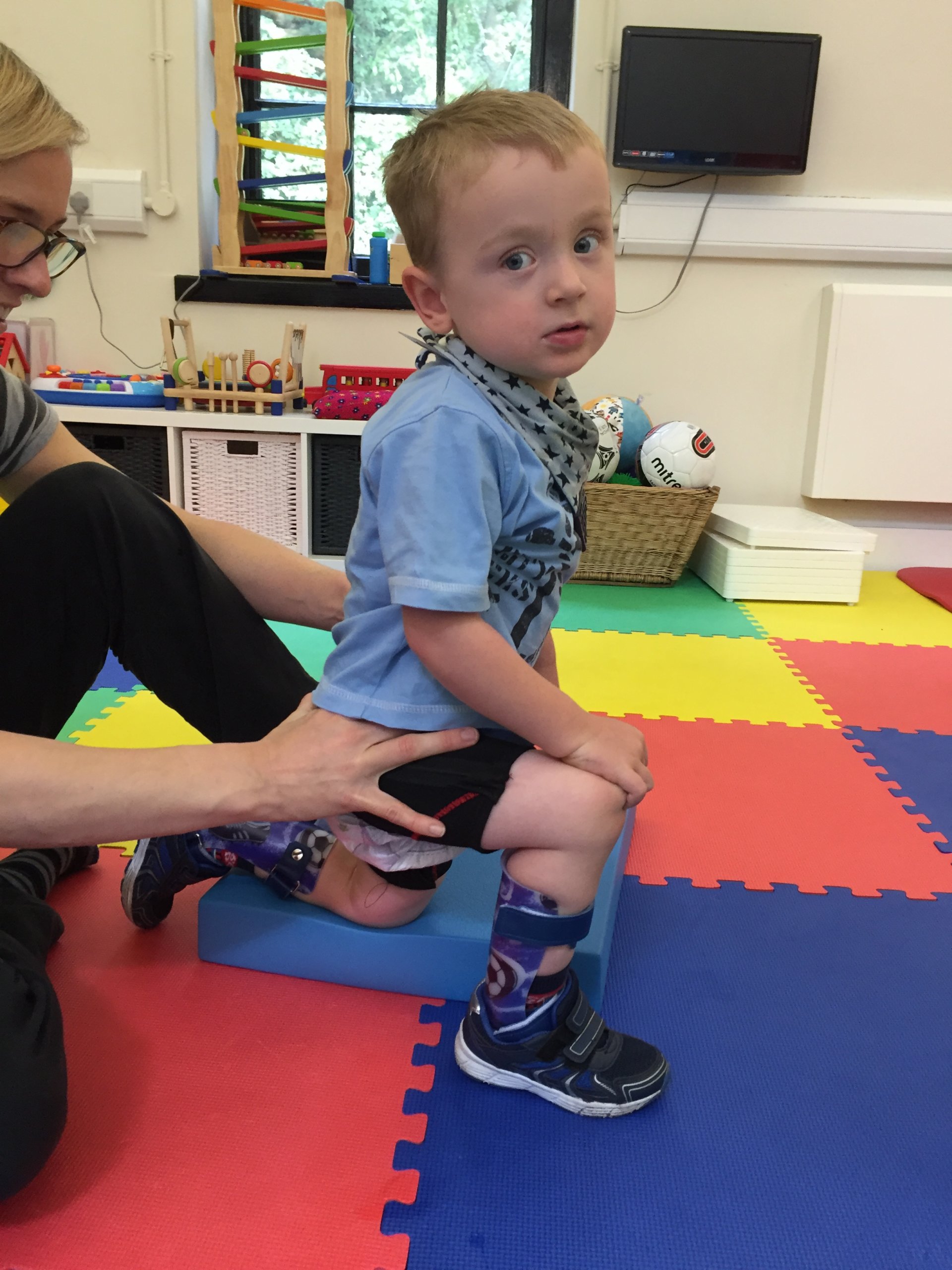The image depicts a cute little boy, approximately five years old, receiving physical therapy in a playroom adorned with a colorful puzzle floor design and scattered toys. The boy, wearing a light blue short-sleeve t-shirt and a stylish scarf reminiscent of a Western sheriff, is kneeling on the floor with braces on both legs near his ankles. His right leg is bent, and he gazes at the camera with a calm, slightly worried expression. Behind him, a smiling woman with glasses and partially blonde hair, dressed in dark pants, supports him at his waist, suggesting she is the therapist administering the treatment. In the background, there is a small TV and various playroom items, which contribute to the warm, nurturing environment.